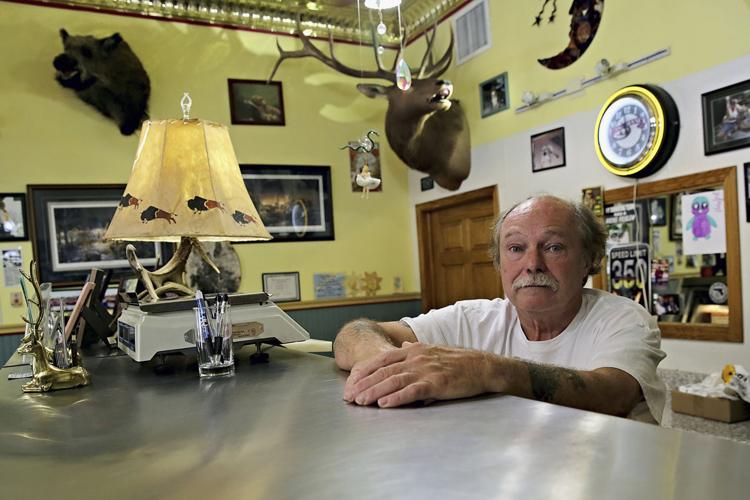In this indoor scene, an older gentleman, likely in his 70s, stands on the right side of the photo, leaning against a high, stainless steel counter. He is partially bald, with gray hair on the sides and a matching gray mustache, and is dressed in a white short-sleeved t-shirt. His arms, displaying some tattoos, rest on the counter, which features various items including a lamp with a base made of deer antlers, a small glass filled with pens, and a measuring scale. 

The setting appears to be a cluttered, almost suffocating man cave or store with walls painted an unappealing yellow. Behind the man are several taxidermied animals, including a boar's head on the top left and a large deer head with impressive antlers in the center. The room also hosts various hunting decorations, picture frames, a mirror, some art pieces, and a clock mounted on the wall.